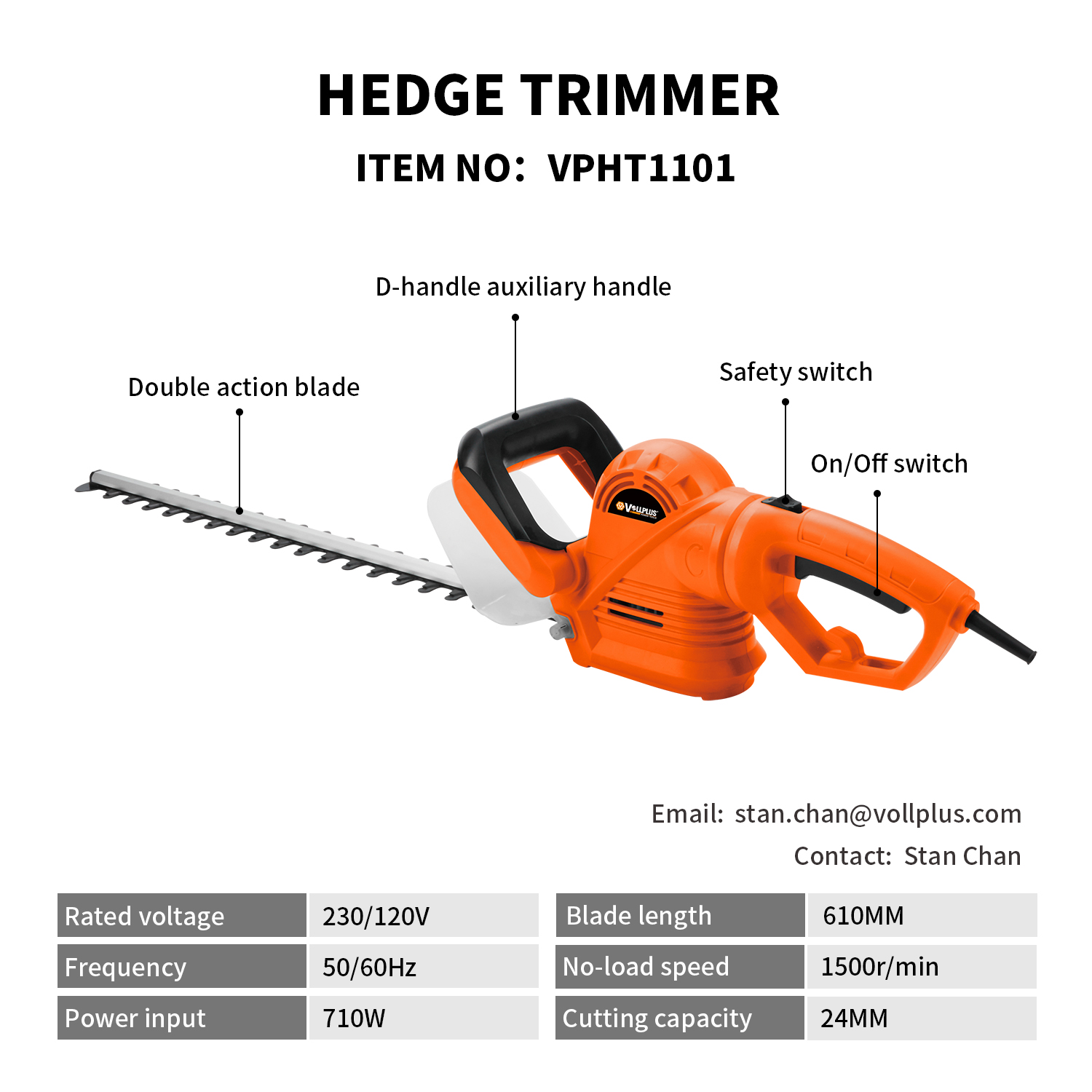This image displays an orange, black, and white hedge trimmer against a white background, prominently labeled "HEDGE TRIMMER" in black uppercase letters across the top, with the item number "VPHT1101" directly below. The trimmer's significant parts are clearly identified with lines pointing to each: the double-action blade, the D-handle auxiliary handle, the safety switch, and the on/off switch. Positioned beneath the hedge trimmer photo is contact information for Stan Chan at VoliPus.com, followed by a detailed specification chart. This chart lists critical technical details, including rated voltage, frequency, power input, blade length, no-load speed, and cutting capacity. The overall layout provides a comprehensive overview of the hedge trimmer and its specifications.